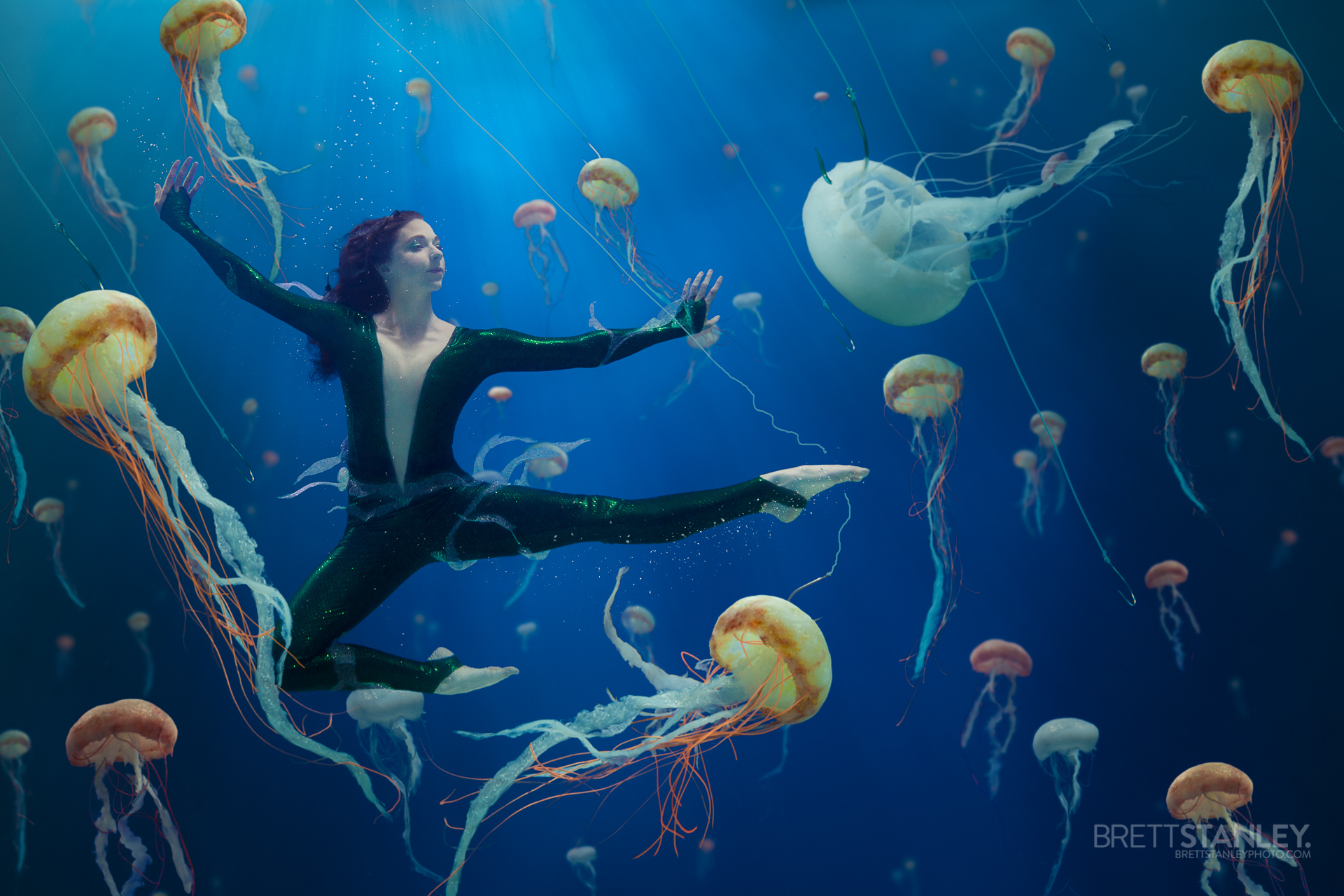This highly detailed image appears to be a digitally manipulated underwater scene, creating an almost surreal visual. At the center-left, an androgynous woman with long dark hair is suspended in a dancer's pose, her body slightly contorted as she kicks outward to the right. She wears a sleek black leotard with a distinctive V-shaped opening stretching from her chest to underneath her groin, connecting to black stirrups over her feet and fingerless gloves, forming an all-encompassing bodysuit. The background is a gradient of blues, darker at the edges and lighter towards the center, evoking the depths of the ocean. Intriguingly, she is surrounded by numerous jellyfish in hues of white, yellow, and orange, some of which are hooked on fishing lines while others drift freely. These hooks are dispersed throughout the image, both with and without jellyfish attached. Light filters down from above, adding to the immersive underwater illusion. Near the bottom right corner, the text “Brett Stanley” appears in a transparent white font, discreetly attributing the artwork to its creator.